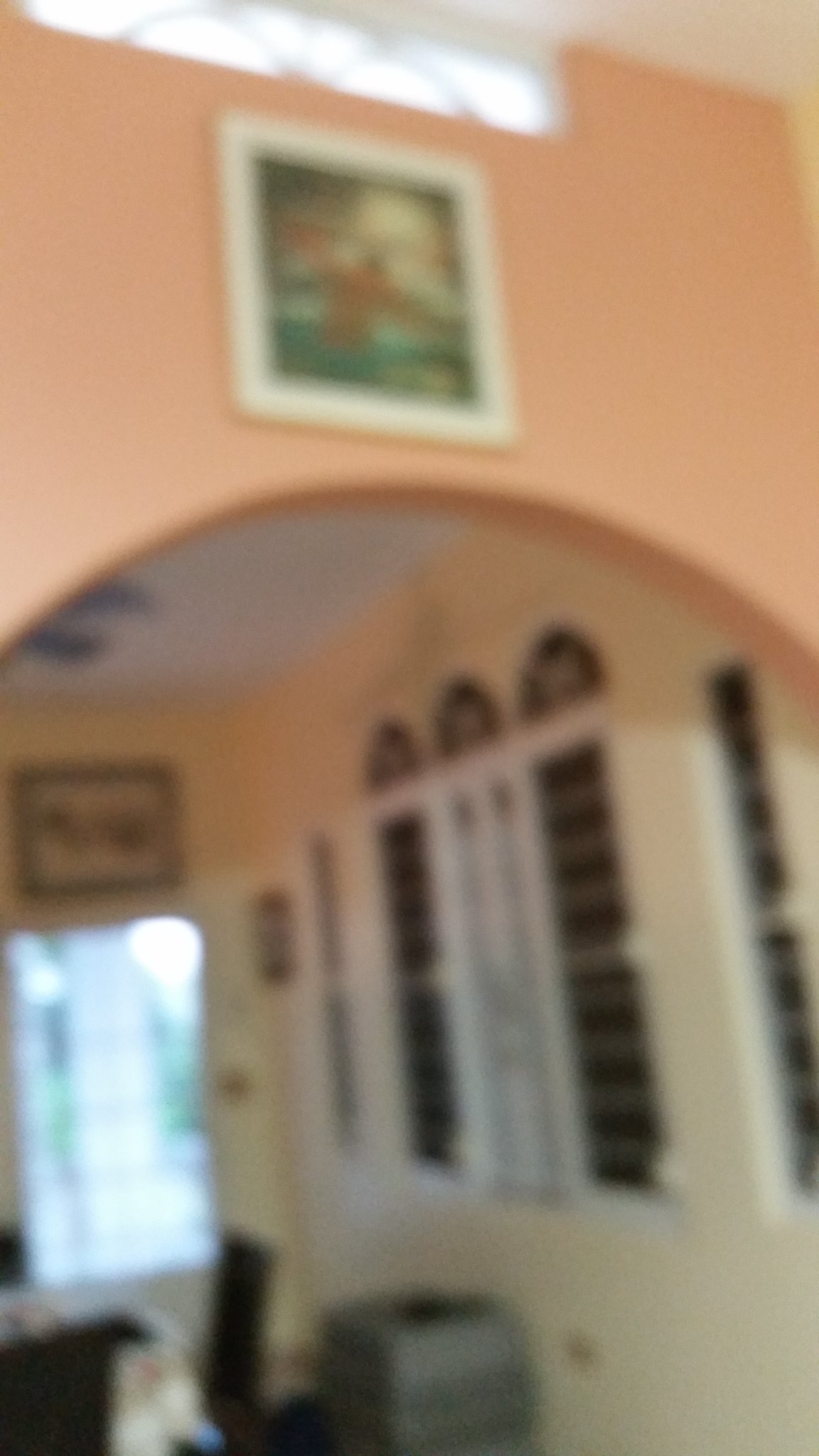This is a blurry image of the interior of someone's house. The focus is on an upper section that includes a unique arched window with an intricate divider. Below this window, there is a peach-colored wall with an arched picture frame mounted on it. Situated beneath the wall, potentially part of a dining or eating area, there are built-in cabinets or shelves, though it's difficult to discern clearly. The shelves appear to have decorative arched plates placed on top. To the right, a door with glass panels allows a glimpse of the bright exterior. Above this door, there is another picture. In the foreground, multiple chairs and a gray object can be seen, suggesting a dining area setup.